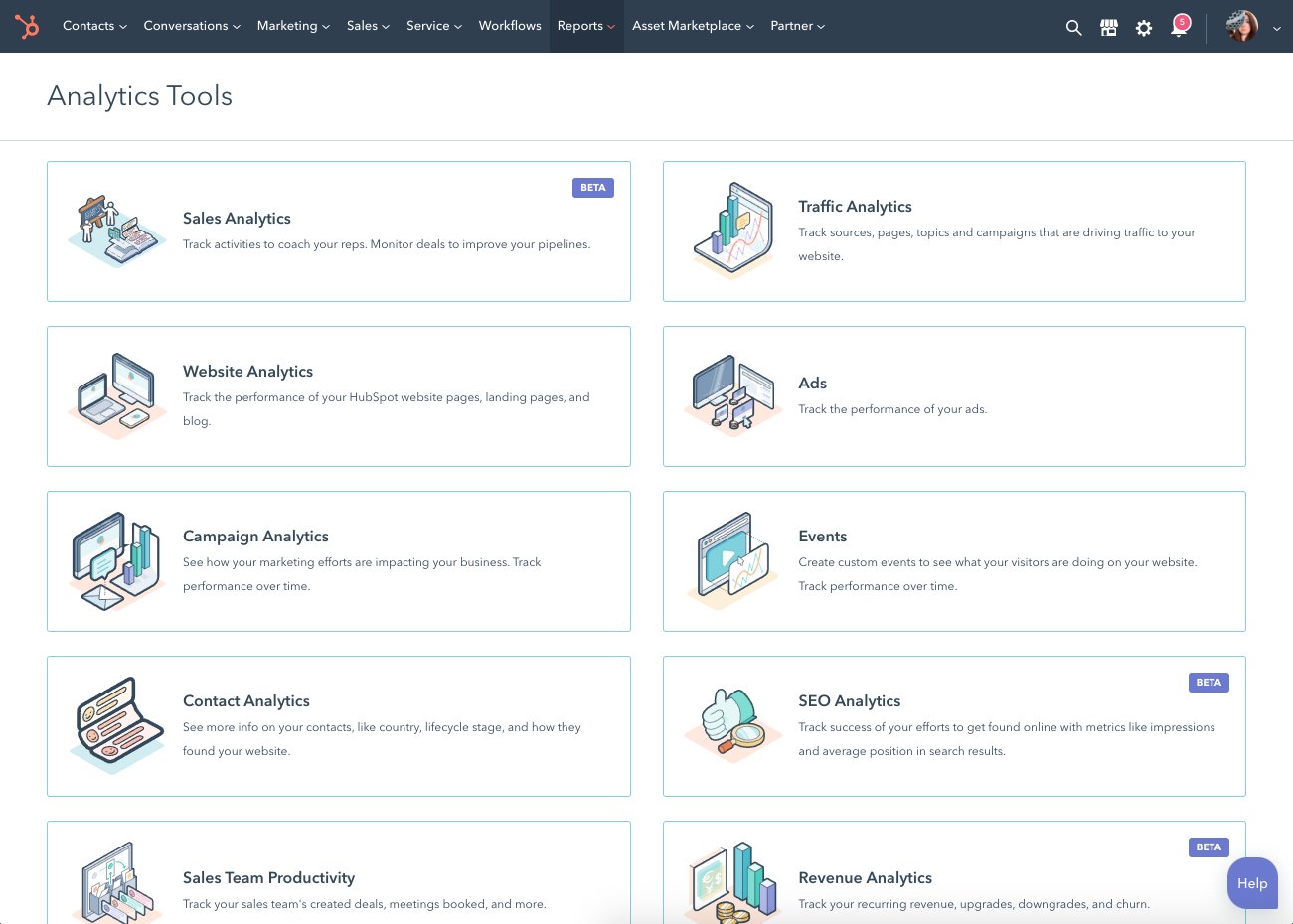This is a detailed screenshot of a dynamic application interface. At the top, there is a dark bluish-gray header bar that spans the entire width of the screen. On the left side of the header, an orange circular logo is visible, characterized by three nodes connected to the circle by thin orange lines, with one node pointing downward to the left, another upward to the left, and the last one pointing directly upward. To the immediate right of the logo, a series of white text labels are present: "Contacts," "Conversations," "Marketing," "Sales," "Service," and "Workflows," almost each accompanied by a white arrow pointing downward except for "Workflows."

Further right, the "Reports" label stands out with an orange arrow pointing downwards and a surrounding dark rectangle highlighting it. Continuing in the same patterned sequence, "Asset Marketplace" and "Partner" appear. There's a section of negative space leading to the right side of the header populated by several icons: a white magnifying glass, a white generic shop icon, a white cog, and a white bell with a noteworthy large pink circle featuring a white numeral '5' outlined in white at the top right.

A vertical white separator line marks the division, followed by a circular profile picture of a woman with brown hair to the right of the line. The profile picture is accompanied by a white arrow pointing downward.

Beneath the header lies the body of the page, set against a white background. In the top-left corner of the body section, "Analytics Tools" is written in large dark gray text. Directly below this heading, a thin light gray line horizontally slices across the entire page. The main content area is structured into rows, each containing two panes. These panes boast a white background bordered by a thin light blue outline. Each pane houses a simple icon on the left side, bold dark gray text adjacent to the icon, and smaller light gray text placed beneath the heading text.